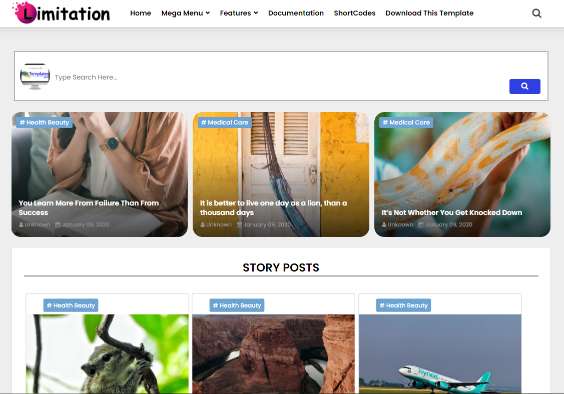This image appears to be a screenshot of a computer screen taken from a website. At the top of the screen, there is a white border with website navigation elements. In the upper left corner, there is a red circle containing the letter "L." To the right of the red circle, the word "Imitation" is displayed. The navigation bar includes options labeled: Home, Mega Menu, Features, Documentation, Shortcodes, Download this Template, and a search icon.

Below the navigation bar is a horizontal gray rectangle. Within this area, there is a white search box that says "Type Search here," accompanied by a typewriter icon on its left and a blue search button on its right.

The main content area features three images arranged horizontally:
1. The first image portrays a female figure with only her arms visible, sitting down. In the upper left corner of this image, the label "Health & Beauty" is displayed.
2. To the right, the second image shows a white door set against a yellow wall. Its upper left corner is labeled "Medical Care."
3. The third image depicts a yellow and white snake wrapped around a branch. Similarly, it is labeled "Medical Care" in the upper left corner. The title accompanying this image reads, "It's Not Whether You Get Knocked Down."

Beneath these images, there is a section titled "Story Posts" which features three additional images:
1. The first picture is labeled "Squirrel on a Branch," showing an image of a squirrel perched on a branch.
2. Next to it, a second picture appears to show a canyon landscape.
3. The final image displays a blue airplane poised for takeoff against a blue sky, suggesting the theme of aviation or travel.